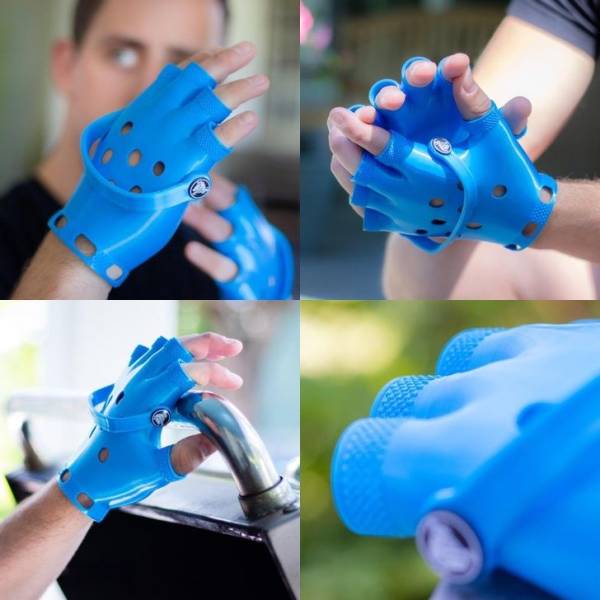The image is a bright, daylight-filled 2x2 grid featuring four detailed photographs of a man showcasing unique blue, fingerless gloves made of a shiny, plastic material reminiscent of Crocs shoes. The gloves feature circular cutouts and a strap-like handle across the knuckles. In the top left photo, the man, dressed in a black t-shirt, holds up both gloved hands prominently. The top right photo focuses on the man's upper body as he sits, his hands held together to emphasize the gloves. The bottom left image captures the man’s left hand wearing the glove, gripping a metal railing. Lastly, the bottom right image provides an extreme close-up of the glove, clearly displaying the circular cutouts and the openings for the pointer, middle, and ring fingers against a green background.